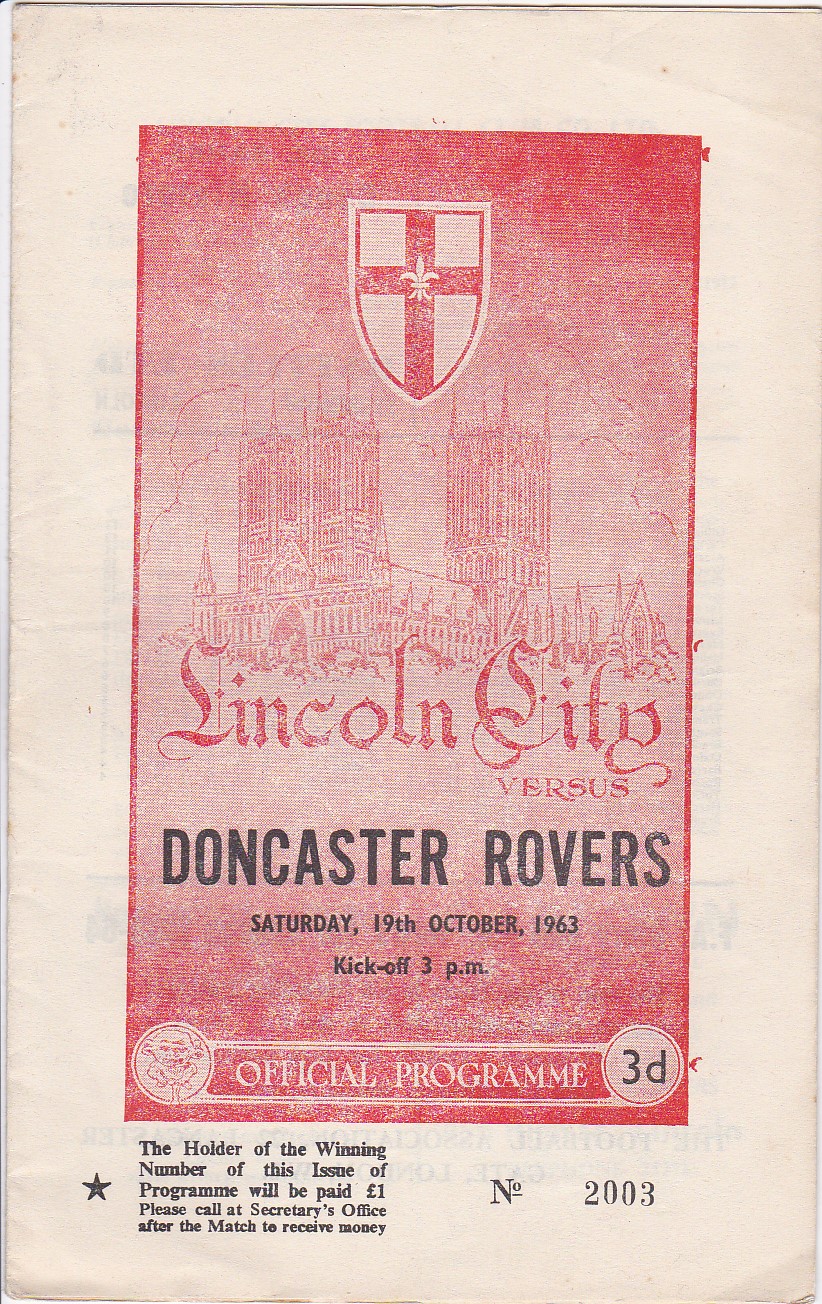The image is the front cover of an official program for a soccer match held on Saturday, October 19th, 1963, with a kickoff at 3 p.m. The design features a white background with an off-white, reddish border on the left. At the top, there's a prominent red and white shield displaying a red cross with a white cross at its center, possibly an emblem. Below, two red-printed buildings, likely depicting a cathedral with two towers, serve as a backdrop for the text. "Lincoln City" is written in red script, followed by "versus Doncaster Rovers" in black print. Further down in smaller red text, the date and kickoff time are provided. The text "Official Program" appears within a rectangular border, with a club symbol to the left and a small circular emblem to the right displaying "3D," indicating the price. The program number "2003" is noted, and a declaration reads, "The holder of the winning number of this issue of the program will be paid one pound. Please call at Secretary's Office after the match to receive the money."